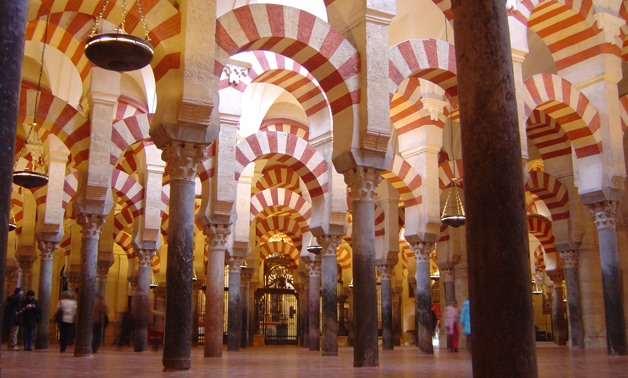This is a highly detailed color photograph of the interior of an ancient, Middle Eastern building, characterized by a striking architectural design featuring a large number of thick cylindrical columns. These columns, likely crafted from stone or a stucco-like material, rise majestically to support intricate arches that span the vast interior space. The arches and columns are decorated in a traditional striped pattern of creamy white and red, which adds to the historical and cultural ambiance of the structure. The alternating colors of the arches create a visually complex and repetitive pattern, with the photograph capturing the presence of possibly 30 to 40 such columns and around 20 grand arches. The lower parts of some columns appear scorched, hinting at a past fire. Sunlight filters through the structure, illuminating the upper sections and creating contrasting shadows. The ground level of the building is dotted with about ten visitors, blurred as they walk, enhancing the sense of the site being a popular tourist attraction. Additionally, chandeliers resembling genie lamps hang from the roof, adding to the antiquated charm of the interior.